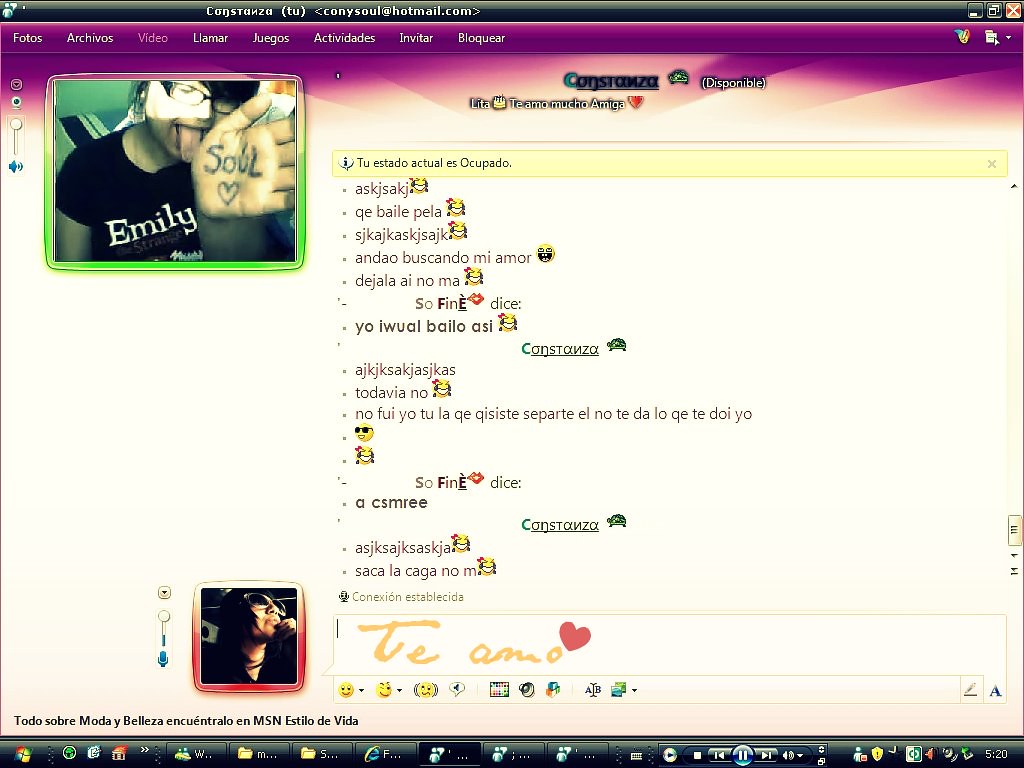The image is a detailed screenshot of an MSN Messenger chat window on a Windows computer. At the very top, there's a black bar featuring a red 'X' for closing the application. The chat appears to involve a user named Constanza, with the email address conysoul@hotmail.com. The interface shows a purple taskbar and all the words are in a foreign language, though the word "video" can be recognized. On the top left, a smaller inset window displays a webcam photo of someone wearing glasses and a black T-shirt with the name "Emily" written in white. This person is licking their hand, which has the word "soul" and a heart symbol drawn on the palm. The main chat section between them and another person is in an unreadable language but resembles a back-and-forth messaging format. In the bottom left corner, another small picture shows a person with shoulder-length dark hair wearing large sunglasses and looking upwards, seemingly taken as a selfie. Additional graphics or stickers in the chat box include something that says "hey mo," which means "I love you." All these combined suggest a snapshot from an active conversation on MSN Messenger, capturing a moment of lively interaction between the two users.